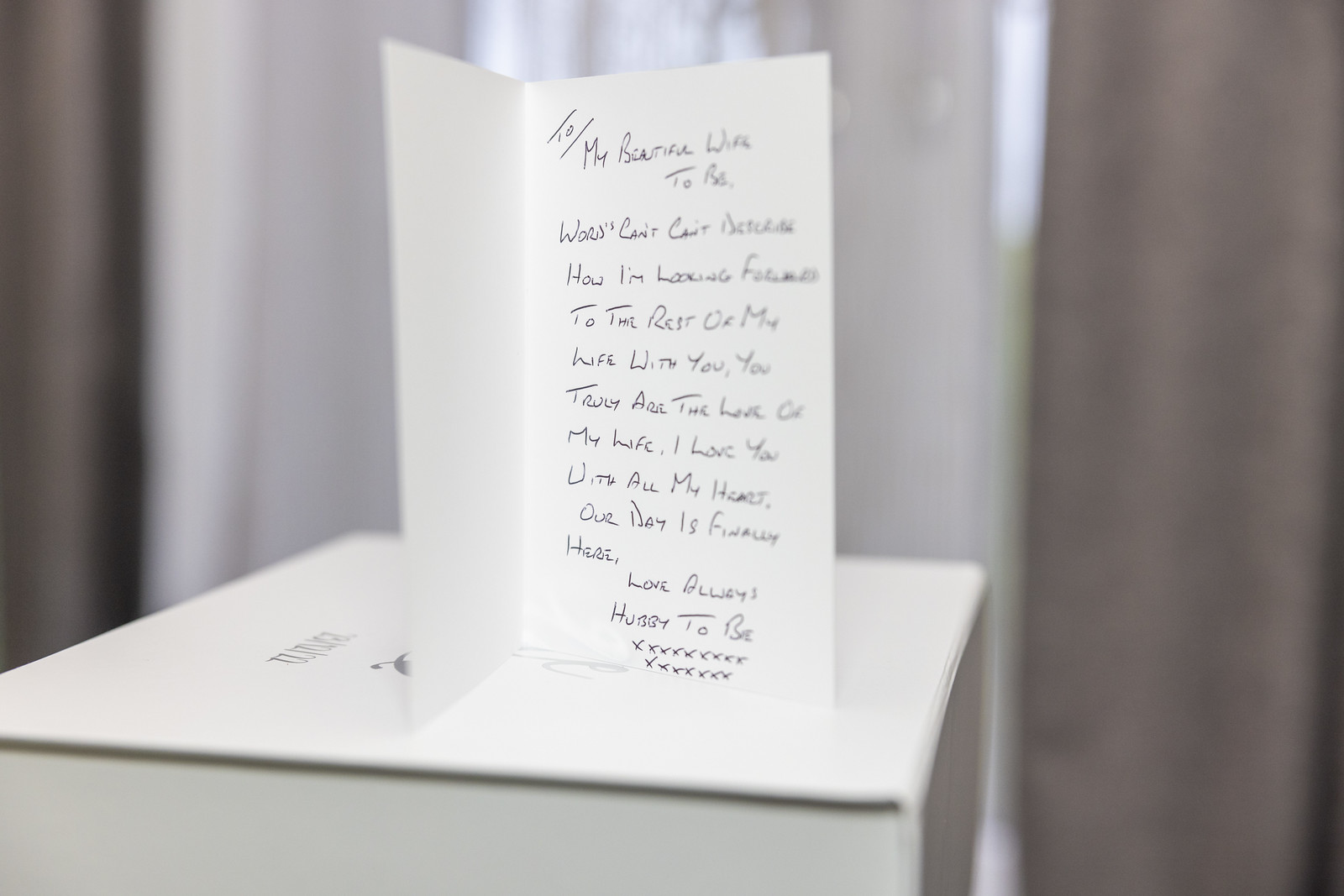The black and white photograph captures a folded card standing upright on what appears to be a white surface. The card, positioned prominently in the center of the image, is the main focal point, while the surroundings—including slightly blurred white and gray curtains in the background—provide minimal context to its setting, possibly an indistinct room. The card is printed and partially handwritten in black ink. The visible text on the card reads: "To my beautiful wife-to-be, words can't describe how I'm looking forward to the rest of my life with you. You truly are the love of my life. I love you with all my heart. Our day is finally here. Love always, hubby-to-be." At the bottom of the card are numerous “x’s,” commonly symbolizing kisses. The neat layout of the text, combined with heartfelt handwritten portions, conveys a deeply personal and sentimental message from a groom to his bride.